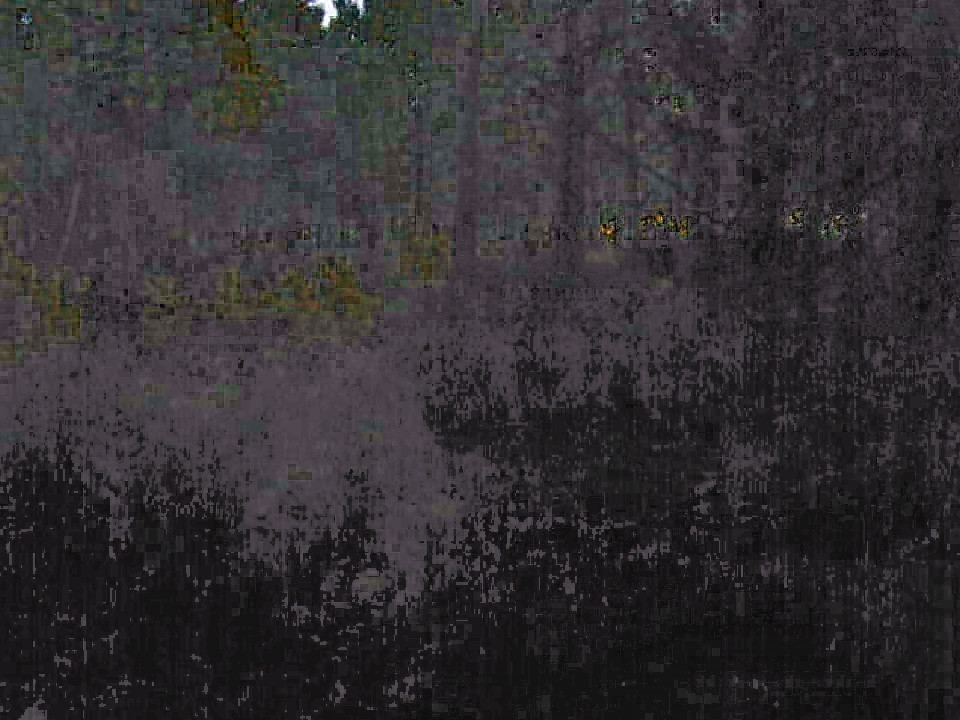The image features a predominantly gray background, transitioning to deep, dark blue and black tones towards the corners and the bottom. The center and upper portions maintain a more consistent gray hue, creating a gradient effect. Scattered throughout are clusters of green foliage punctuated by yellow dots, possibly indicative of blossoming flowers or illuminated leaves. The overall composition is somewhat indistinct and fuzzy, evoking an abstract representation of a dark, dense forest with shadowy trees and ambiguous forms that might resemble roots or underbrush.